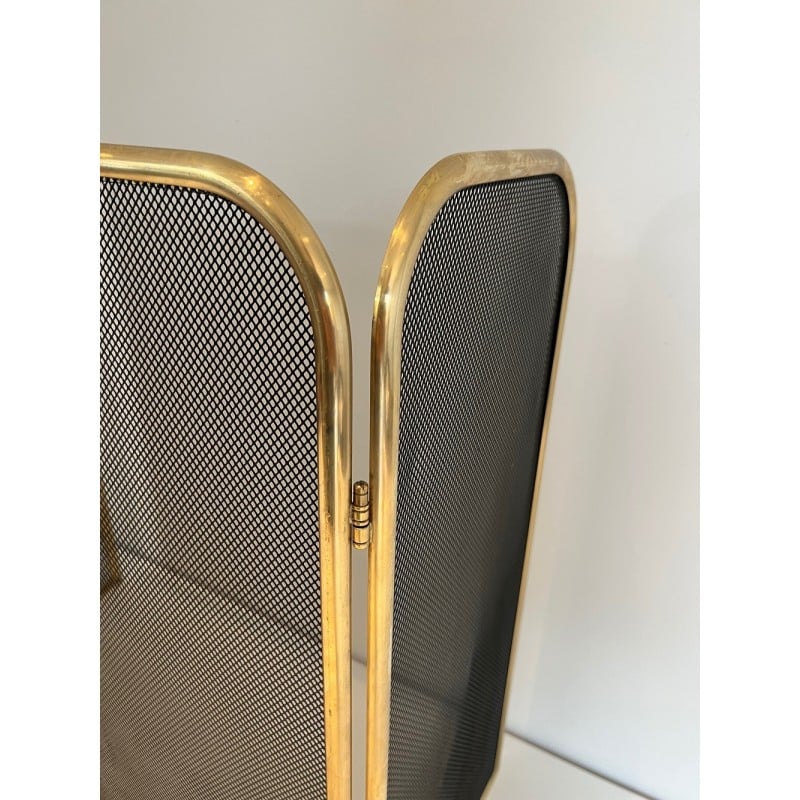A striking gold floor gate with a black mesh center stands prominently against a pristine white floor. The gate's elegant design features a gleaming gold metallic trim that complements its sturdy construction. Positioned to enclose a specific area, this gate is likely intended to prevent pets from accessing certain sections of the home. The surrounding walls on the right are painted a crisp white, accentuating the gate's luxurious appearance. Every element in the image is aligned perfectly, contributing to a sense of order and functionality.